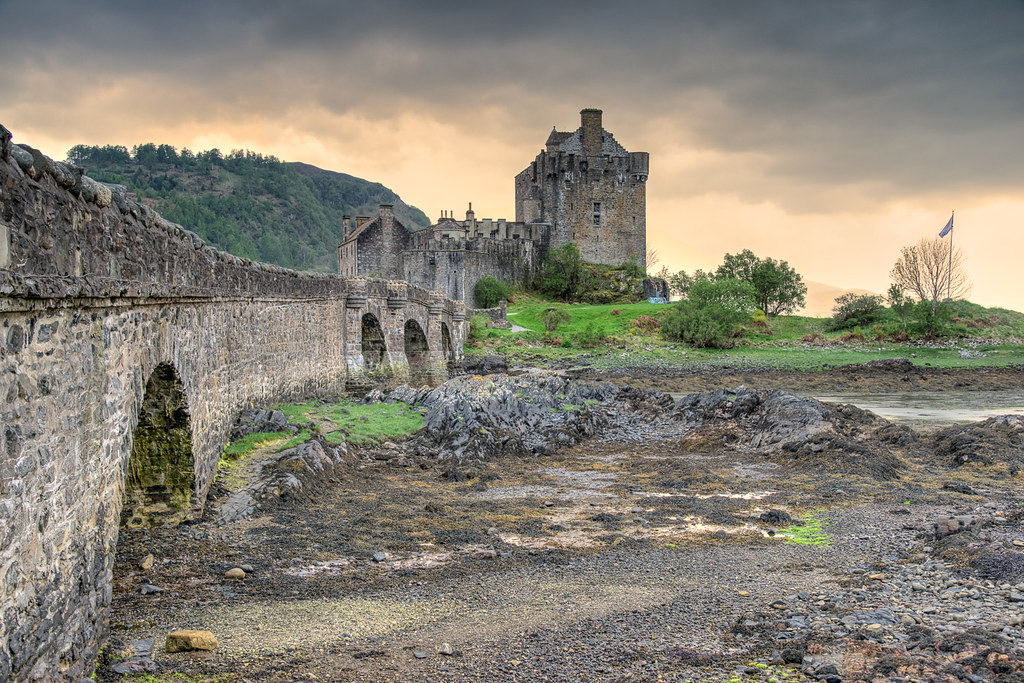The image is a full-color, horizontally rectangular photograph taken outdoors on a very gloomy, overcast day. It depicts a large, ancient castle made of grey stone, identifiable as a medieval monument. Leading to the castle is an old stone bridge with arches, spanning over a rocky, unkempt terrain with patches of grass, gravel, and occasional shrubs and small trees. The lower half of the image showcases this rugged landscape, while a small, seemingly dried-up body of water is visible nearby. Toward the center-right, there's a flag fluttering on a pole. The entire scene is set against a backdrop of dark grey clouds, adding to the ominous atmosphere. A hill-like structure is noticeable on the left side of the image. The castle, reminiscent of grand estates such as Downton Abbey, stands as a testament to affluent medieval architecture.